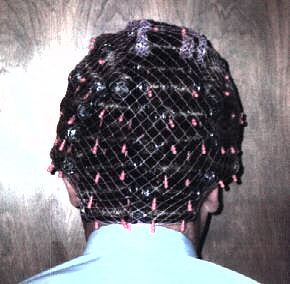The image is a small, square photograph that focuses on the back of a person's head as they face a dark wood-paneled wall. The muted, muddy colors of the image are disrupted by a large glare coming from the left-hand side, likely caused by the camera flash. The person's black hair is pinned up in various curlers and secured with pink, horseshoe-shaped pins under a silver hairnet. They are wearing a light blue collared shirt, visible from the top of the back just below the neck to where the picture cuts off before reaching the shoulders. The tightly pinned and curled hairstyle suggests that the person is either in the process of having their hair done or has recently styled it.